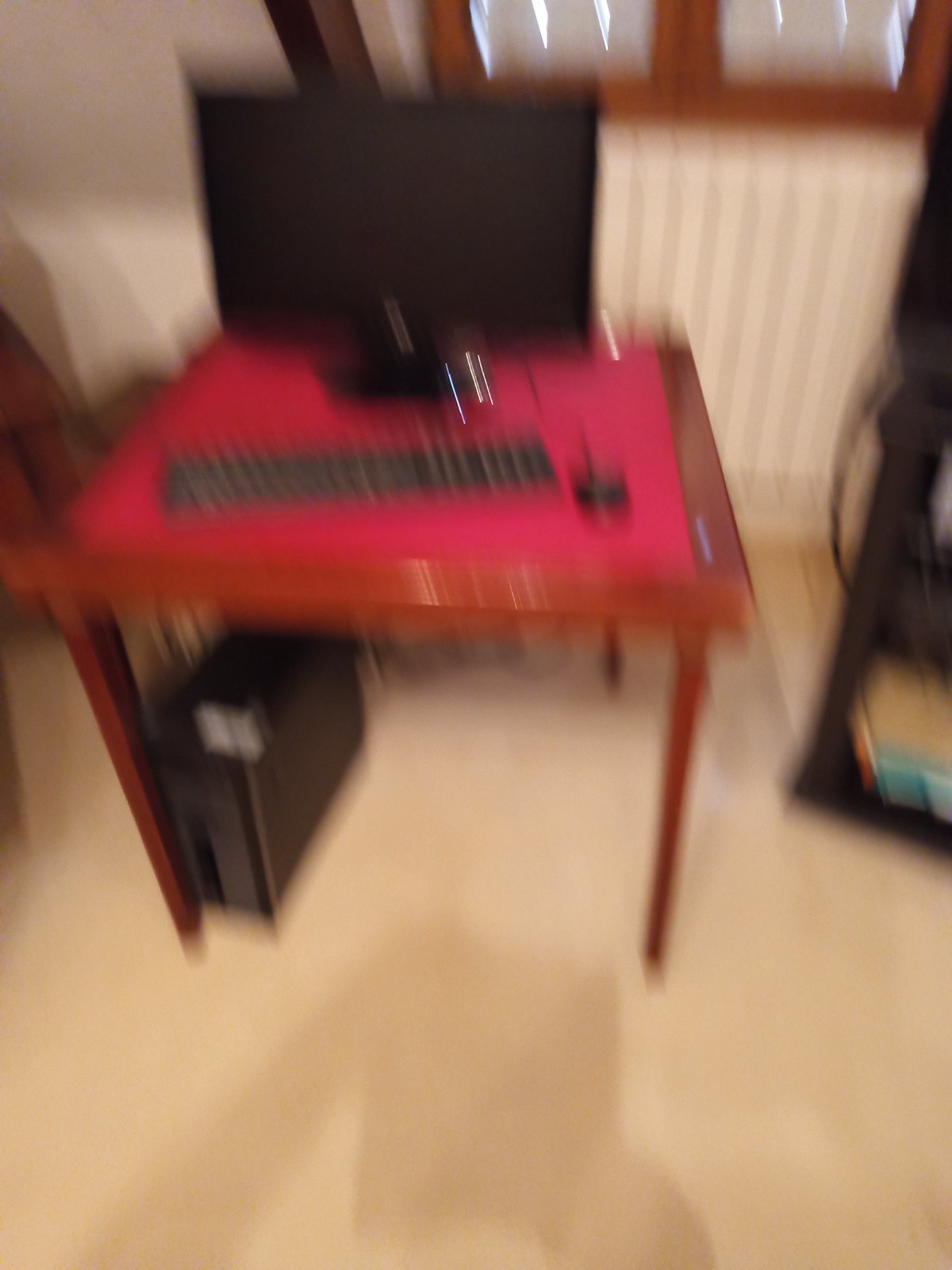This very blurry photograph depicts a front view of a setup with a brown wooden table, covered by a red mat or cloth. On the table sits a black computer monitor with its screen turned off, a black keyboard with white lettering, and a black mouse. Underneath the table, on the left-hand side by the left leg, there's a black computer tower. The setup appears to be placed on a tan-colored floor, with a white radiator against the wall behind it. Above the radiator is a window or a cabinet with a wooden frame, though the blurriness makes it indistinguishable. The wall itself has vertical white slats, contributing to the room's somewhat bright atmosphere. No chair is present in the scene, further enhancing the minimalist appearance of the workspace.